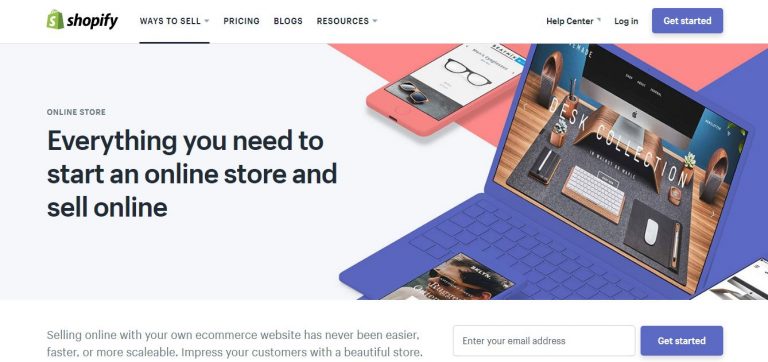The image is a rectangular advertisement or website layout for Shopify, oriented with the longer side extending horizontally. In the upper left-hand corner, there is a green shopping bag icon with an 'S' on it, labeled "Shopify." The navigation menu includes links for "Ways to Sell," "Pricing," "Blogs," and "Resources." Adjacent to these, on the right side, there are links for the "Help Center" and "Login," followed by a prominent blue button with white text reading "Get Started." This entire section is set against a white background.

Further down, the next section features a large rectangular image depicting a laptop and a cellphone placed on a counter. On the left side of this section, there is text that reads: "Online Store: Everything you need to start an online store and sell online." Below this image, a statement says, "Selling online with your e-commerce website has never been easier, faster, or more scalable. Impress your customers with a beautiful store." Additionally, there is an input box for an email address next to another blue "Get Started" button with white text.